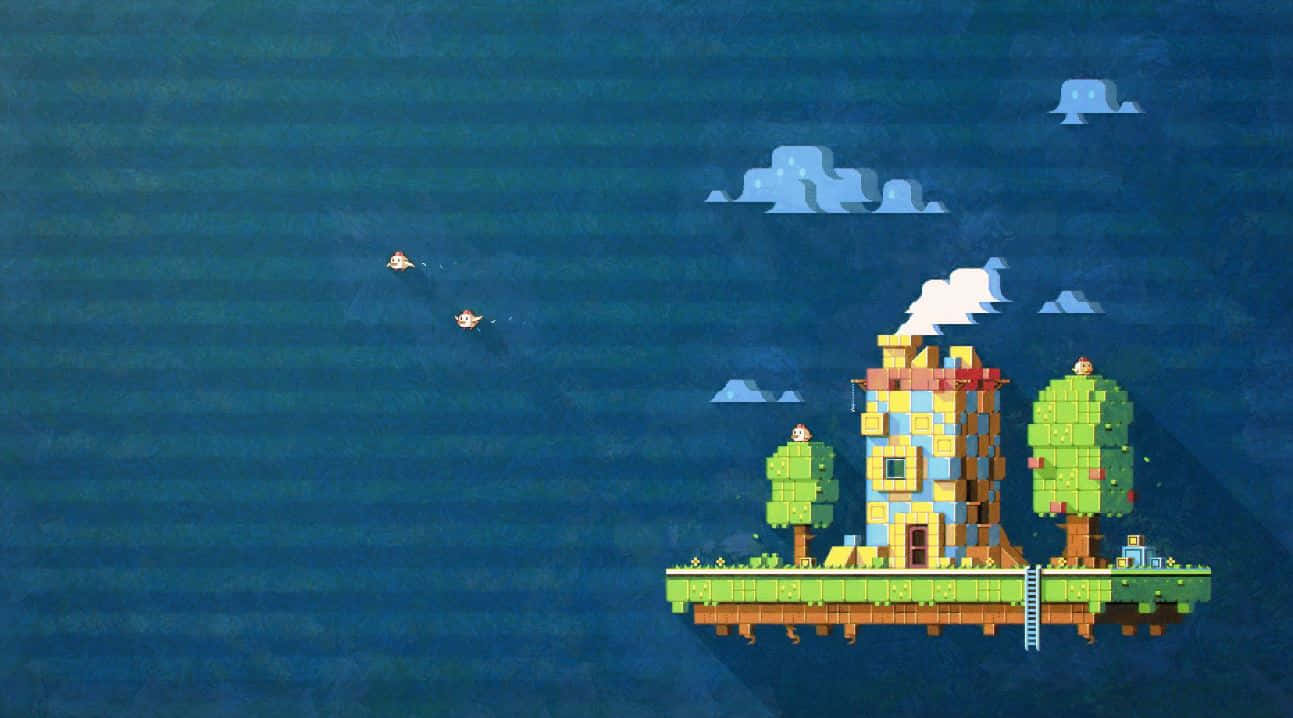The image appears to be a pixelated screenshot reminiscent of a video game, possibly resembling Minecraft or Lego. Central to the scene is a small floating sky island set against a predominantly blue background that evokes a body of water or ocean. The right side of the island features a house characterized by light blue, yellow, and red hues, with smoke billowing from its chimney. Surrounding the house are two trees - one with red apples, complemented by birds perched atop it. A ladder extends from the house, connecting the ground area, which is covered in green grass and appears to be suspended in the air, exposing some brown earth beneath. Additionally, there are a few crates near the apple tree. Above the scene, pixelated light blue clouds float, and birds are seen flying to the left, enhancing the detailed and whimsical atmosphere of this floating island paradise.